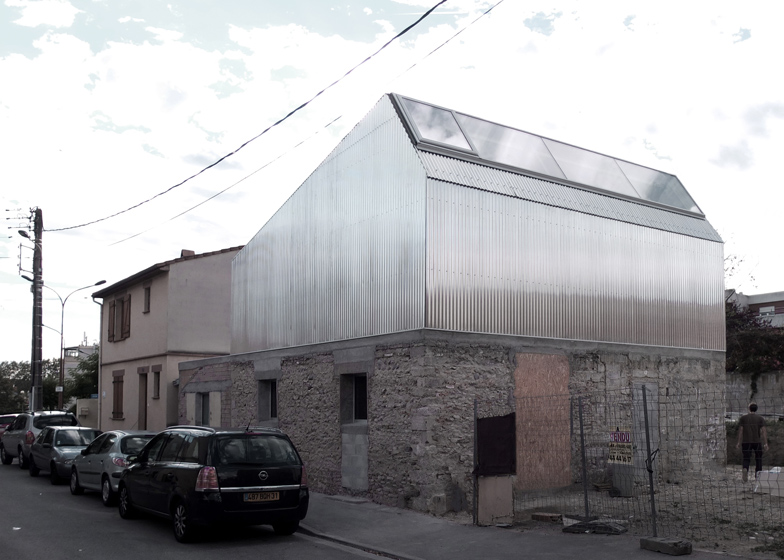The photograph captures a sunlit, outdoor setting with a variety of detailed features. On the bottom left, a road lined with parked vehicles leads the eye towards a gray concrete sidewalk on its right. The sidewalk is accompanied by an electrical pole with extending power lines. Adjacent to the sidewalk, a row of houses stands prominent. The house closer to the left is painted in light beige with dark brown accents, while the house further right has a distinctive design. This house features a stone-brick ground floor, and its upper floor appears to be constructed from metallic or silver material, giving it a greenhouse-like appearance with clear plastic or glass windows allowing sunlight to permeate. In the bottom right corner, a tall, metal wire fence encloses a space where a man stands with his back to the camera, seemingly gardening with others in a dirt area. Above, the sky is a mix of bright blue and white clouds, adding to the overall clarity and brightness of the scene. The image is sharply clear, with natural light enhancing the visibility of its varied elements.